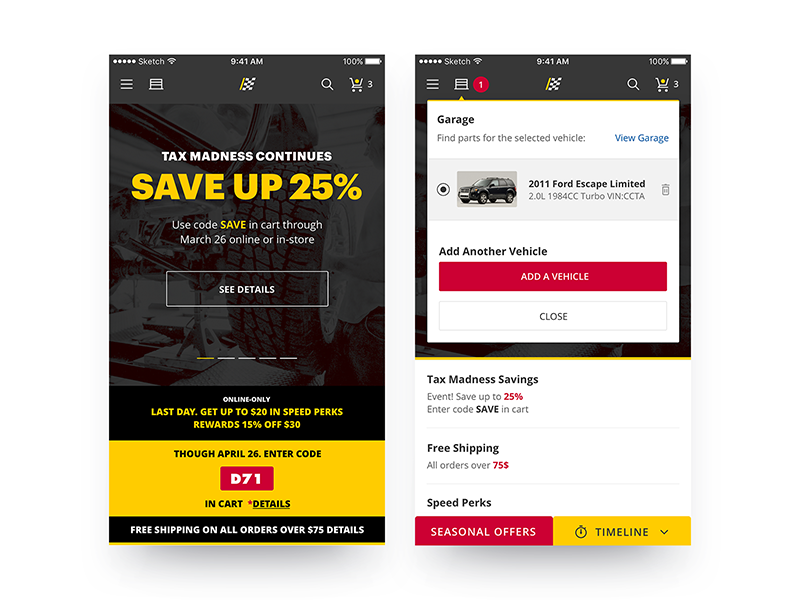This pair of screenshots, both taken at 9:41 a.m. with 100% battery life, showcase a promotional advertisement with multiple elements. The top section features a navigation bar that includes a hamburger menu icon, a search icon (magnifying glass), and a cart icon with a yellow circle indicating the number "3."

The main promotional text, styled in bold yellow lettering, announces: "Madness Continues. Save Up to 25%." Additional details clarify, "Use Code SAVE," applicable both online and in-store through March 26. There is a call-to-action button in a white box labeled "See Details."

Below this primary promotion, there are five horizontal gray dashes, with the first one colored in yellow, indicating some form of progress or selection. A secondary offer highlights an "Online Only" deal stating: "Last Day, Get Up to $20 in Speed Perks Rewards 15% Off $30," valid through April 26. The promo code "D71" is featured in white text on a red rectangle, accompanied by another call-to-action button labeled "Details" on a black rectangle.

Both screenshots also mention, "Free Shipping on All Orders Over $75," and provide details for further information. In the second screenshot, the navigation bar slightly differs by displaying three rectangles instead of a magnifying glass.

This detailed visual representation aims to entice customers to take advantage of multiple promotions, clearly outlining the discounts, promo codes, and terms for both online and in-store purchases.